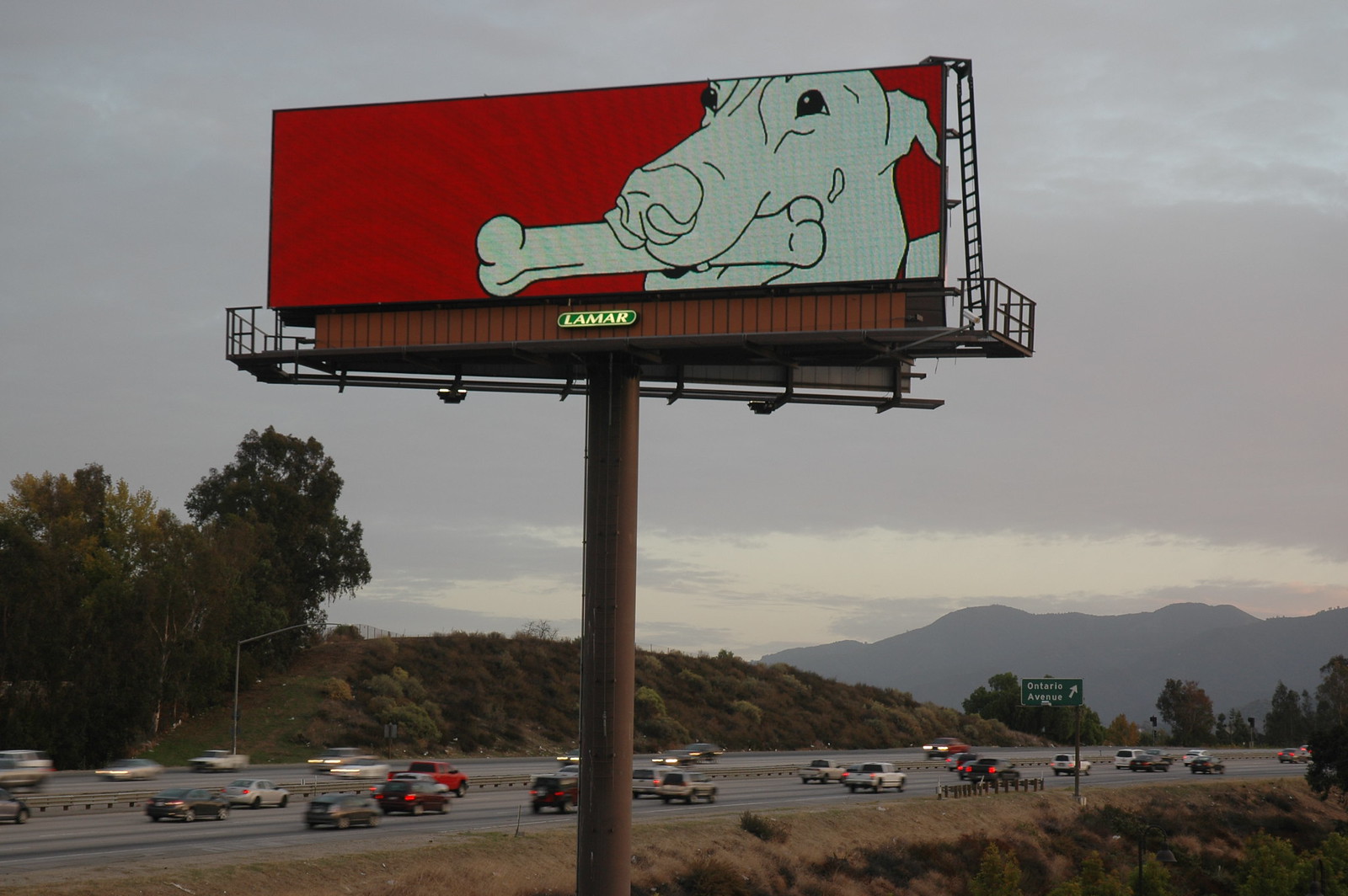The photograph captures a vivid billboard atop a dark brown support post, towering over a multi-lane highway. The rectangular billboard, set against a striking red background, features a black and white illustration of a dog gripping a bone in its mouth. The dog, characterized by a long nose, short hair, and dark eyes, commands attention. Below, the busy highway is visible with numerous cars traveling in both directions. In the bottom right corner, a green road sign indicating "Ontario Avenue" with an arrow pointing to the top right is noticeable. Beyond the bustling roadway, a range of mountains stretches across the horizon under a cloudy, gray sky, adding depth and context to the scene.